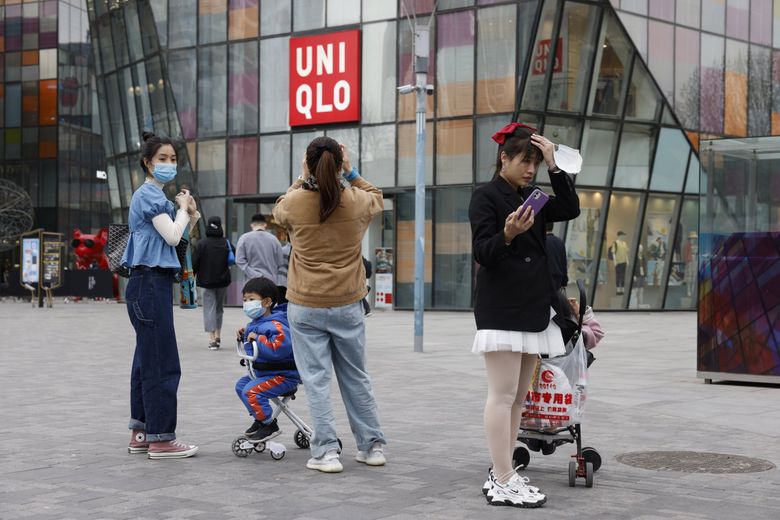The photo captures a bustling city courtyard lined with various storefronts, prominently featuring a large Uniqlo store distinguished by its big red logo affixed against a building with numerous windows of different colors. The space is pedestrian-only, free of cars, and paved with stone, measuring about twice the width of a typical roadway, suggesting a dedicated shopping area. In the foreground, several younger to middle-aged Asian pedestrians, most donning COVID masks and dressed in long sleeves appropriate for cooler weather, occupy the scene. On the left, a lady in a blue blouse and jeans, holding a bag and a mask, looks towards another woman who is facing the Uniqlo store and taking a photo. Between them stands a child in an orange and blue sweatsuit. Additionally, a woman dressed in a black jacket and pink skirt, carrying a bag or a cart, is seen taking a selfie. The background showcases a tall building with four visible stories of windows directly ahead and additional stories, possibly eight or nine, extending off to the left.